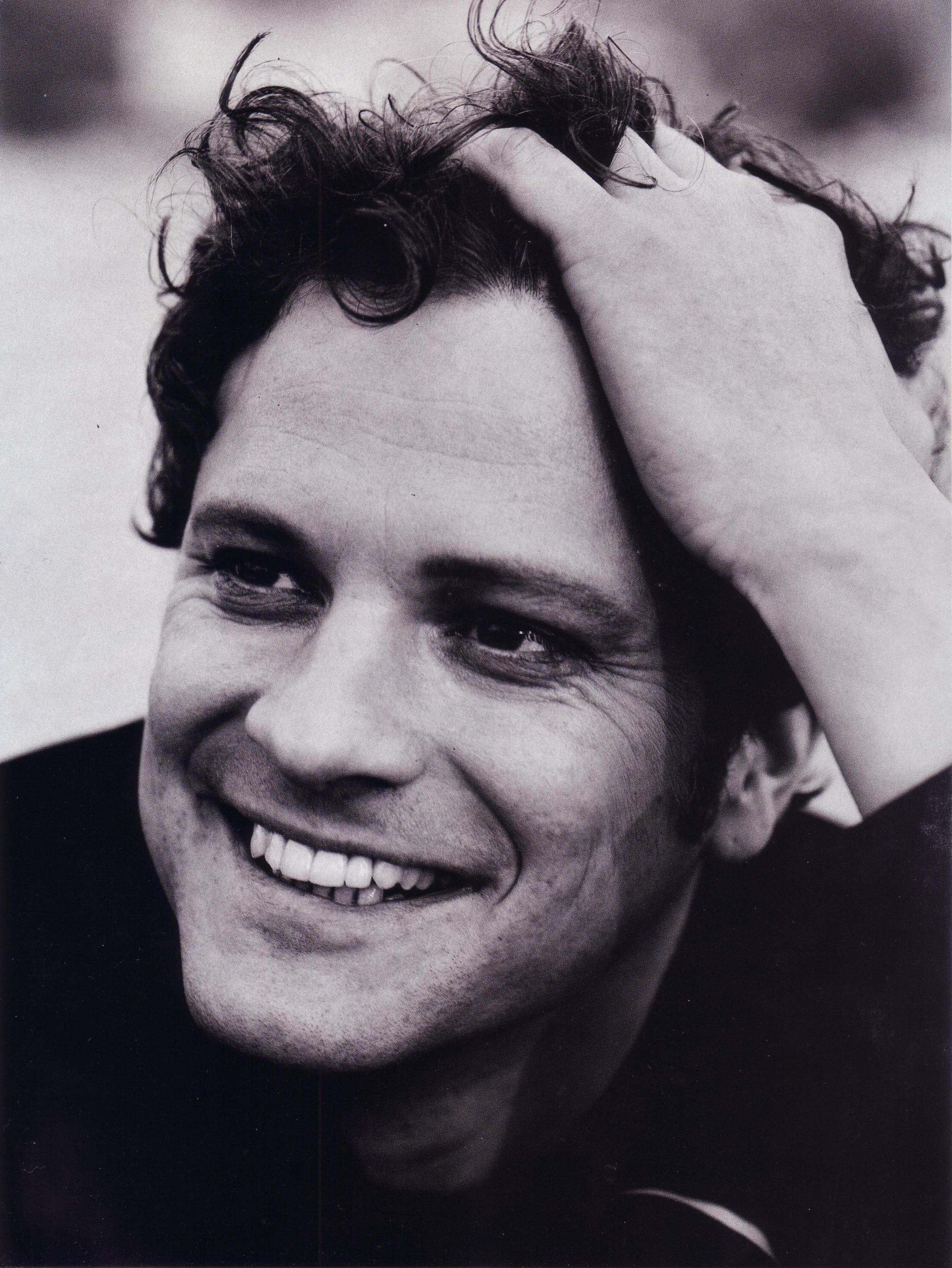This black and white photograph features a close-up of a seemingly youthful Colin Firth, a British actor who appears to be in his 30s or early 40s. The image is centered on Colin's face, capturing him from the neck up with slight visibility of his shoulders, suggesting he is wearing a dark, long-sleeved shirt. His short, dark hair appears slightly curly and somewhat tousled as he runs his left hand through it. Colin's face, adorned with dark eyes and eyebrows, shows a bright, engaging smile, revealing his white teeth. His expression is lively, with noticeable laugh lines around his eyes and grooves near his mouth, indicating genuine joy. He gazes off to the side, and is clean-shaven with a hint of stubble. The blurred and indistinct background consists of grayscale shades, adding depth without distracting from his vibrant expression.